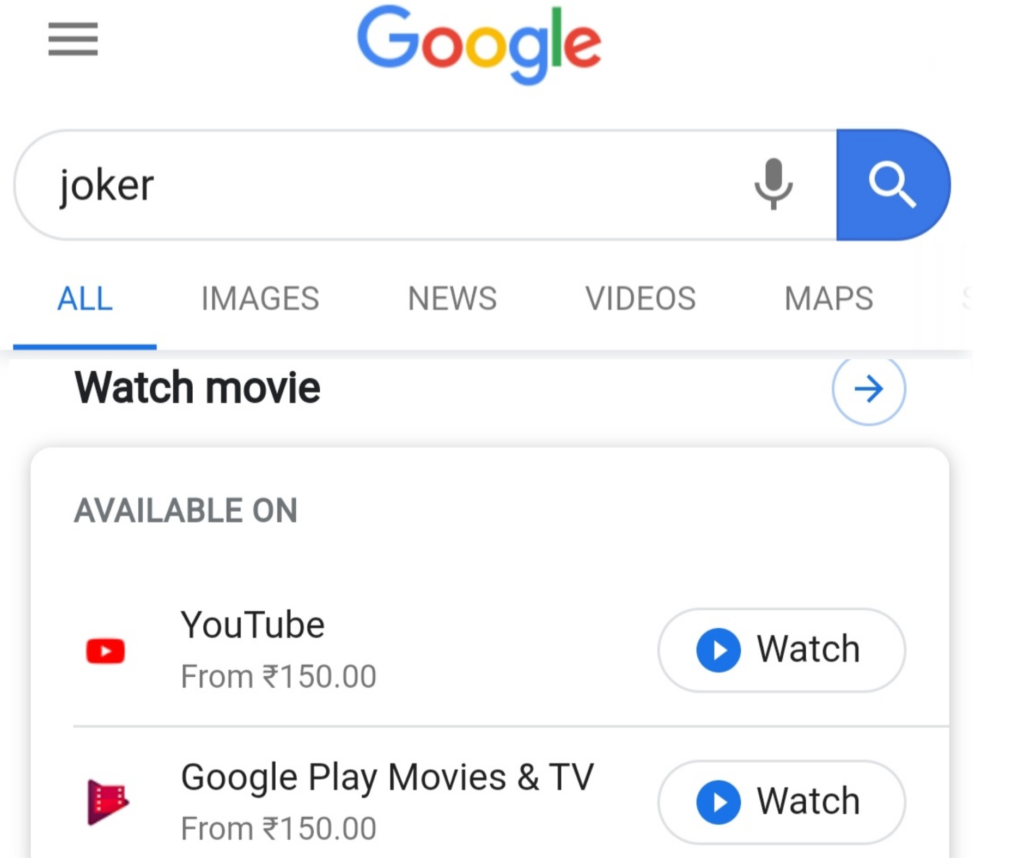**Detailed Screenshot Description:**

The screenshot depicts a smartphone or tablet's display with a Google search interface. At the top, the Google logo is prominently centered, showing a capitalized blue "G," followed by lowercase letters: a red "o," an orange "o," a blue "g," a green "l," and a red "e." To the left of the logo, there are three black horizontal lines.

Beneath the logo, there is an oval search bar with a thin dark gray border. Inside the search bar, bold black text reads "Joker." Next to this text is a microphone icon, which consists of a filled-in upside-down "C" with a line through it. At the right end of the search bar, there is a dark blue microphone icon adjacent to a white magnifying glass icon.

Below the search bar are several navigation tabs. The first tab, labeled "All," is selected and highlighted with a dark blue underline and dark blue text. The subsequent tabs, labeled "Images," "News," "Videos," and "Maps," are displayed in dark gray text.

Following these tabs, bold black text states "Watch Movie." To the right, there is a white circle with a dark blue border and a blue arrow inside pointing right.

Further down, within a rounded rectangle, dark gray all-caps text reads "AVAILABLE ON." Below this heading, a red square with a white right-pointing triangle symbolizes YouTube. Adjacent black text spells out "YouTube" with a capital "Y," followed by lowercase "o," a capital "T," then "ube." The word "From" appears in gray text underneath, displaying an unrecognized currency symbol followed by "150, 150."

To the right, an oval button with a thin gray border contains a blue circle with a right-pointing triangle and bold black text reading "Watch." A similar button appears for another listing, which on the left features a maroon triangle and a red square. Bold black text reads "Google Play Movies & TV," followed by "From 150" with the same unrecognized currency symbol.